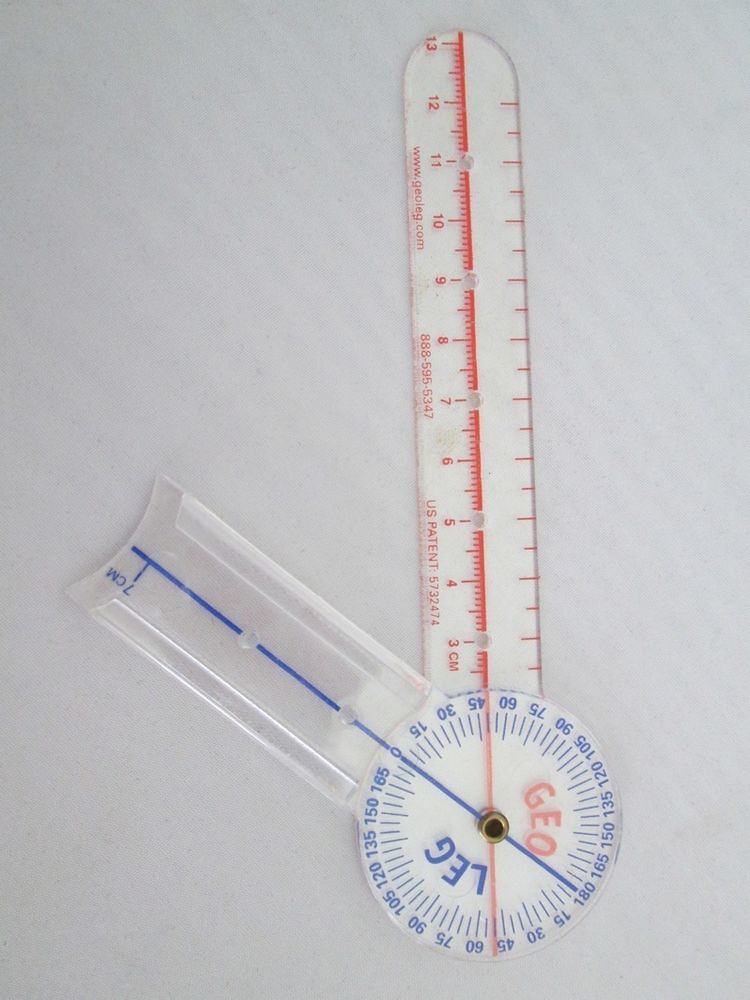An image depicts a precision measuring tool, likely constructed from either plastic or acrylic material, with an overall see-through quality. The tool features two arm-like components, reminiscent of clock hands. The shorter arm, extending to the left, is colored blue and white, whereas the longer arm, stretching upwards, is red and white. Both arms are anchored at a central circular hub, which is detailed with words and numbers. The numbers are arranged in a circular fashion along the edge of this hub, indicating measurement units, while the words "LEG" in blue and "GEO" in red are prominently displayed in capital letters. The background is a simple white surface, providing no additional context or labeling to clarify the specific use of the apparatus.